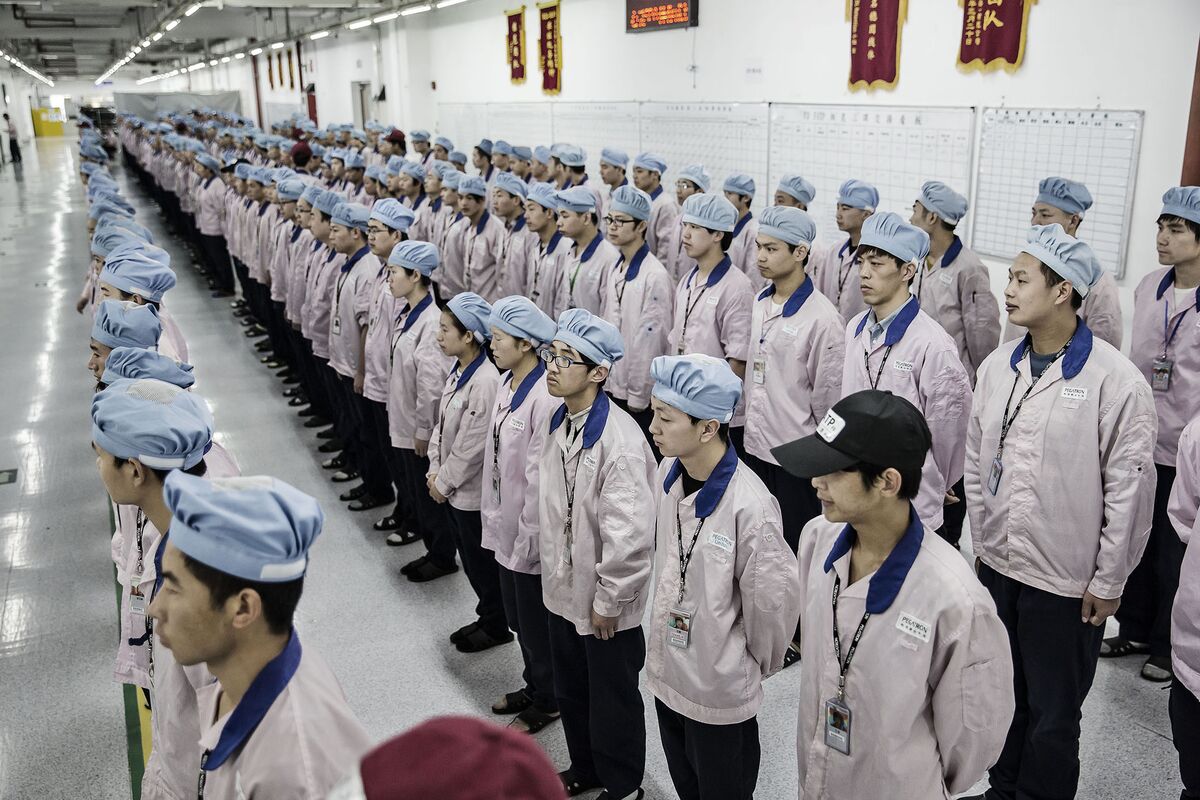This detailed color photograph, in landscape mode, captures a large group of over 100 individuals, appearing to be of Asian descent. They are organized in four neatly aligned rows, all facing towards the front of what seems to be a large, well-lit indoor space, possibly a warehouse or school. Each person is dressed identically in long-sleeve light pink jackets with dark blue collars, black pants, and black shoes. They all wear blue puffy caps, except for a few individuals near the ends, one of whom is wearing a dark baseball cap. Around their necks, they all have lanyards with ID badges featuring their pictures. The scene suggests a uniformity that implies they might be workers or students. In the background, faintly visible are various boards with grids, charts, and banners in red and yellow, possibly bearing Asian writing and signs indicative of either instructional material or organizational insignia.